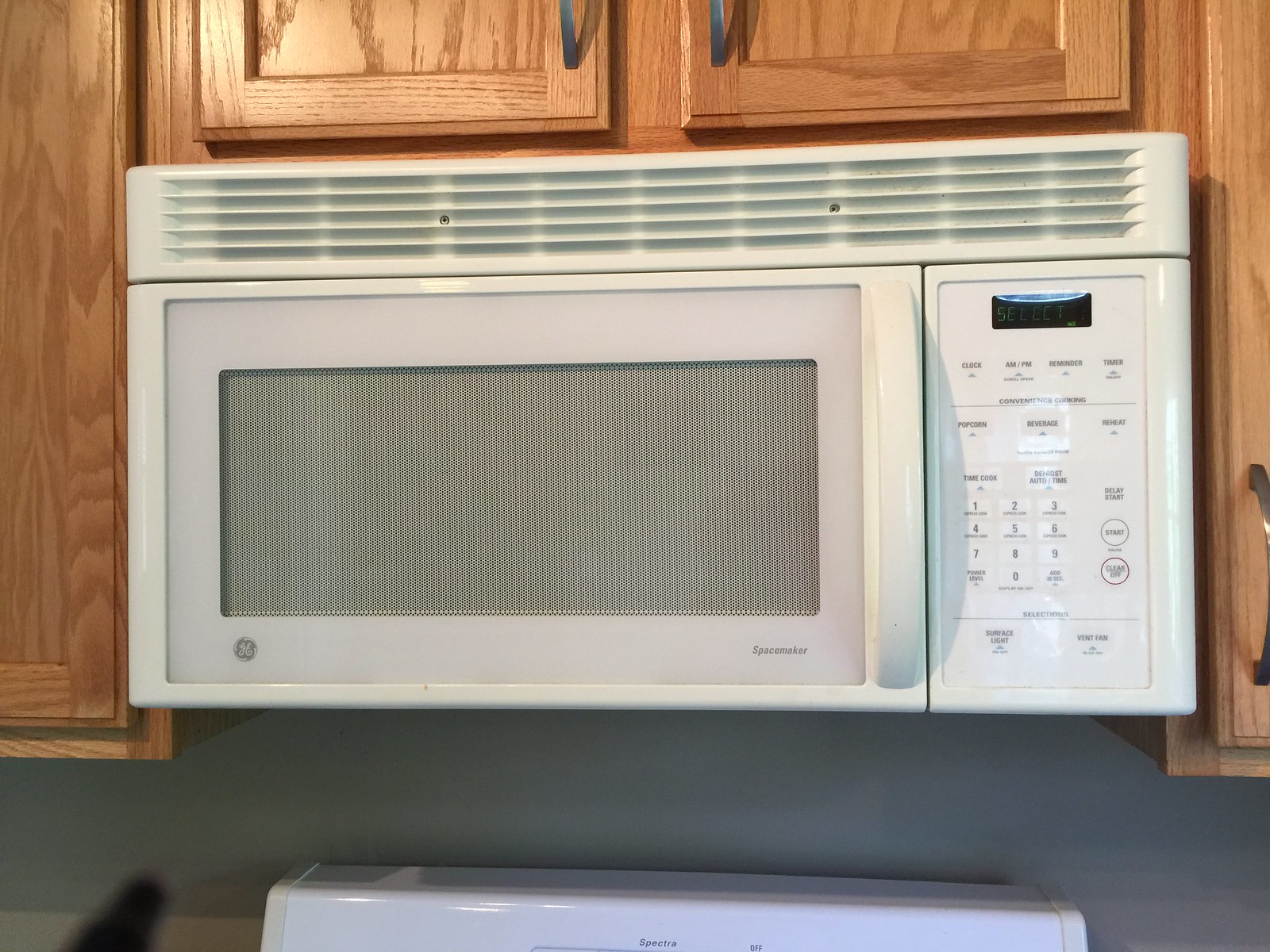The image captures a white GE microwave integrated into a kitchen setup, aligned seamlessly with the surrounding brownish cabinets. The microwave, featuring a handle on the right side designed to be pulled with the left hand, showcases a series of buttons and a digital screen on its right for various settings like warming and defrosting food. Above and around the microwave, there are three visible cabinets with silver handles—two above and one on the right side. The bottom-left cabinet handle is not visible in the frame. The aqua-colored wall behind the microwave adds a touch of color, contrasting with the grayish-blue wall. Below the microwave, the top part of a stove and oven combo peeks into the frame. Additionally, subtle shadows indicate reflections of other kitchen elements, enhancing the depth of the image. The microwave also has ventilation slats on top, ensuring proper airflow.